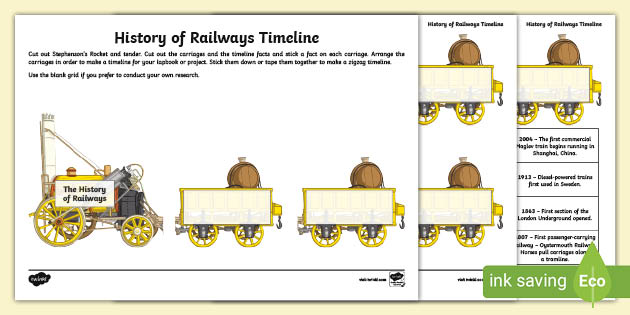This vibrant, colorized illustration, set against a white background and framed by a yellow border, showcases a detailed "History of Railways Timeline." In the top left-hand corner, the heading is rendered in bold black lettering. Beneath the heading, a brief, small-font description likely provides context for the depicted scenes. The illustration features an old-fashioned railway train with yellow wagon wheels, comprising an engine and several carts, some of which carry barrel-like objects. The wheels and carts are unhooked but equipped with latches for potential connection.

The image appears to be part of an educational set, possibly flashcards detailing various stages in railway history. An eco-friendly "ink-saving" label is marked by a green banner with the word "ECO" and a decorative leaf motif in the bottom right-hand corner. Vertically arranged on the far-right and left sides are additional train graphics and timelines. These sections contain columns with historical annotations and illustrations, including one with a notable historical figure. Framed timeline descriptions, presented in black writing within separate boxes, further enrich the understanding of railway evolution. This detailed, folding chart likely serves as an educational tool available from office supply or school supply sources.